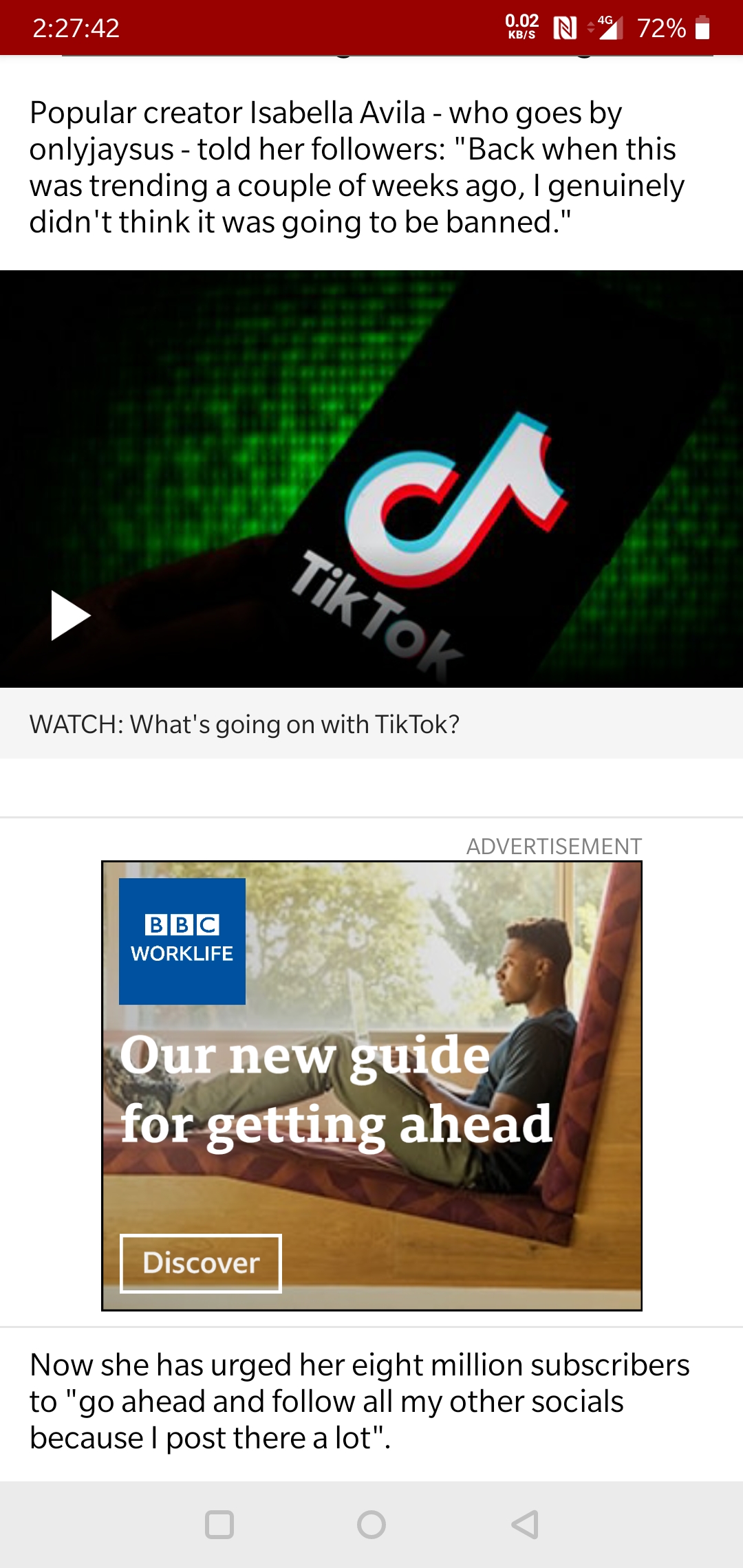This screen capture from a news website offers a detailed overview of the latest trending topic concerning TikTok. At the very top of the screen, a maroon red bar extends across the page. The left side of the bar displays the date, "2-27-42," while the right side shows the current time, a symbol, a Wi-Fi icon indicating a 72% connection, and a battery icon.

Below this bar, the headline reads: "Popular Creator Isabelle Avila, known as only Jsus, sold her followers," hinting at a past event that gained traction a few weeks ago. The caption proceeds with a quote from Avila expressing disbelief over the platform's impending ban: "I genuinely didn't think it was going to be banned."

The image features a person holding a cell phone, displaying the TikTok symbol prominently. Just beneath this, there's a small play button, inviting users to "Watch: What's going on with TikTok?" Directly below this segment, an advertisement for BBC WorkLife appears, promoting a new guide titled "Our New Guide for Getting Ahead."

In the lower section of the screen, there's a "Discover" heading. At the very bottom, a message from Isabelle Avila reads: "Now she has urged her 8 million subscribers to go ahead and follow all my other socials because I post there a lot."

Overall, the image effectively conveys a series of updates and reactions surrounding the potential ban of TikTok, focusing on the actions and advice given by notable creator Isabelle Avila.